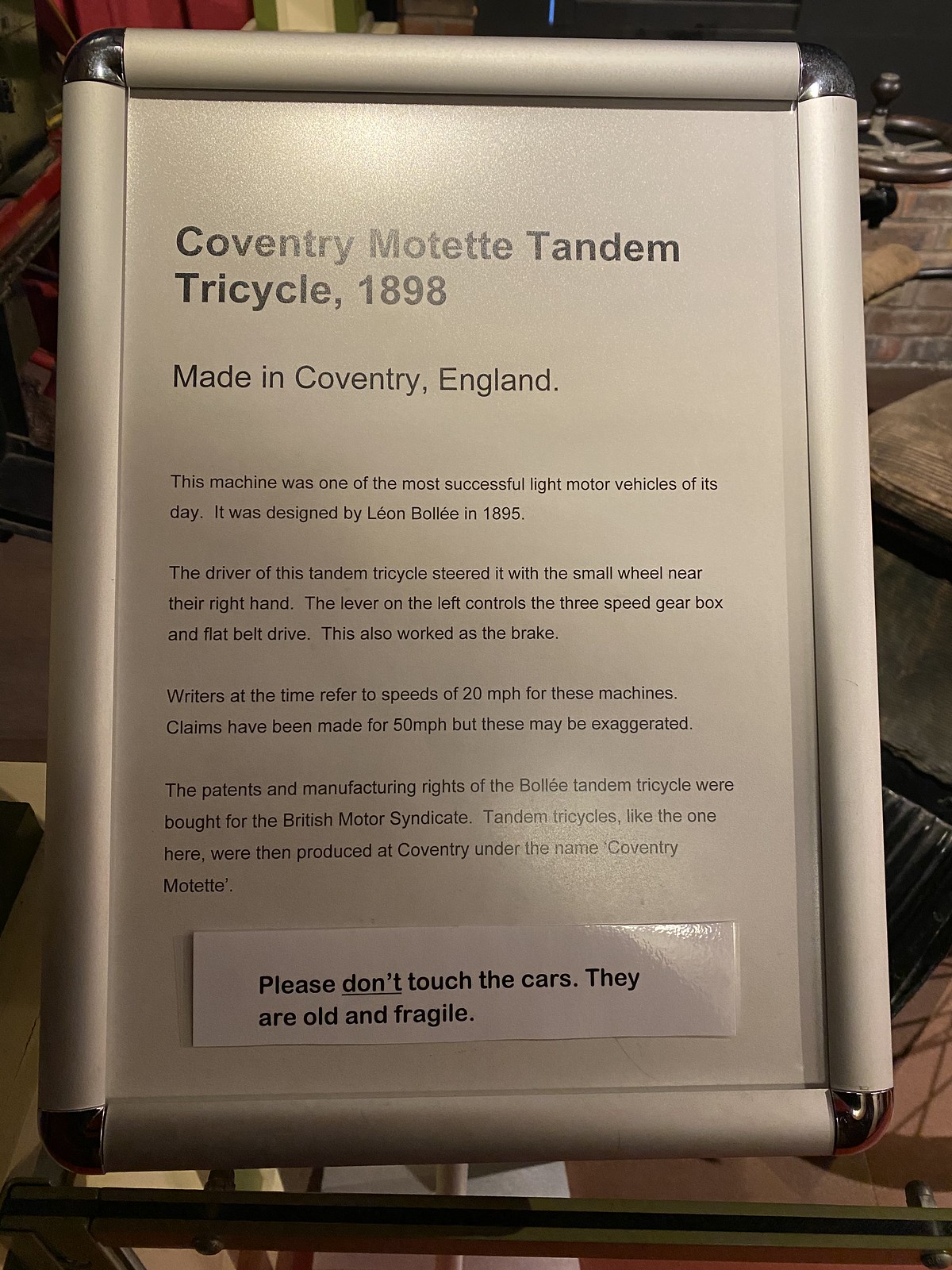The image depicts an information display sign at a museum, framed with silver tubing and shiny chrome corners. The sign itself is flat white with black text, detailing the Coventry Motet tandem tricycle, 1898, made in Coventry, England. It states that this machine was one of the most successful light motor vehicles of its day, designed by Léon Bollée in 1895. The driver steered with a small wheel near their right hand, while a lever on the left controlled the three-speed gearbox and flat belt drive, which also functioned as a brake. Riders at the time reported speeds of up to 20 miles per hour, with some claims of 50 miles per hour likely being exaggerated. The patents and manufacturing rights of the Bollée tandem tricycle were acquired by the British Motor Syndicate, leading to production in Coventry under the name Coventry Motet. Additionally, a plastic insert on the sign warns visitors, "Please don't touch the cars. They are old and fragile."